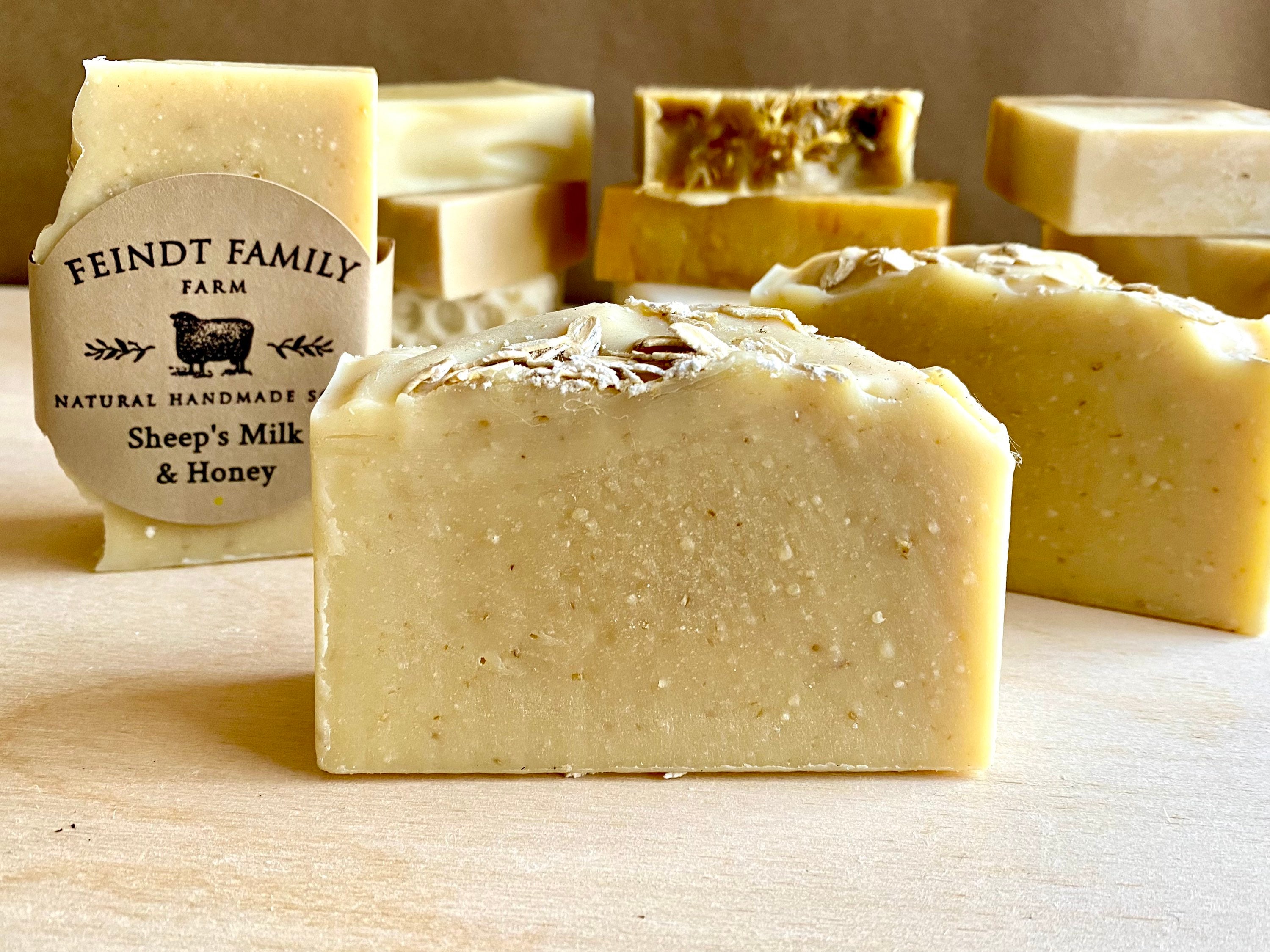This photograph showcases a selection of handmade soaps from Feindt Family Farm, a small business specializing in natural handmade soap using sheep's milk and honey. The soap featured prominently in the foreground is a large, chunky piece with visible oatmeal or similar ingredients on top, highlighting its artisanal texture. On the left side, one soap bar is wrapped in brown paper bearing the Feindt Family Farm logo, which includes a sheep graphic and black lettering stating "natural handmade soap, sheep's milk and honey." The background reveals an assortment of 11 different soap bars in various shapes and sizes, ranging from smooth to coarse textures, and colors from off-white to brownish tones. These soaps, with their rustic, non-uniform appearance, suggest a handcrafted process typical of products found at farmers' markets. The soaps are displayed on a pink surface, emphasizing their artisanal and homemade qualities.